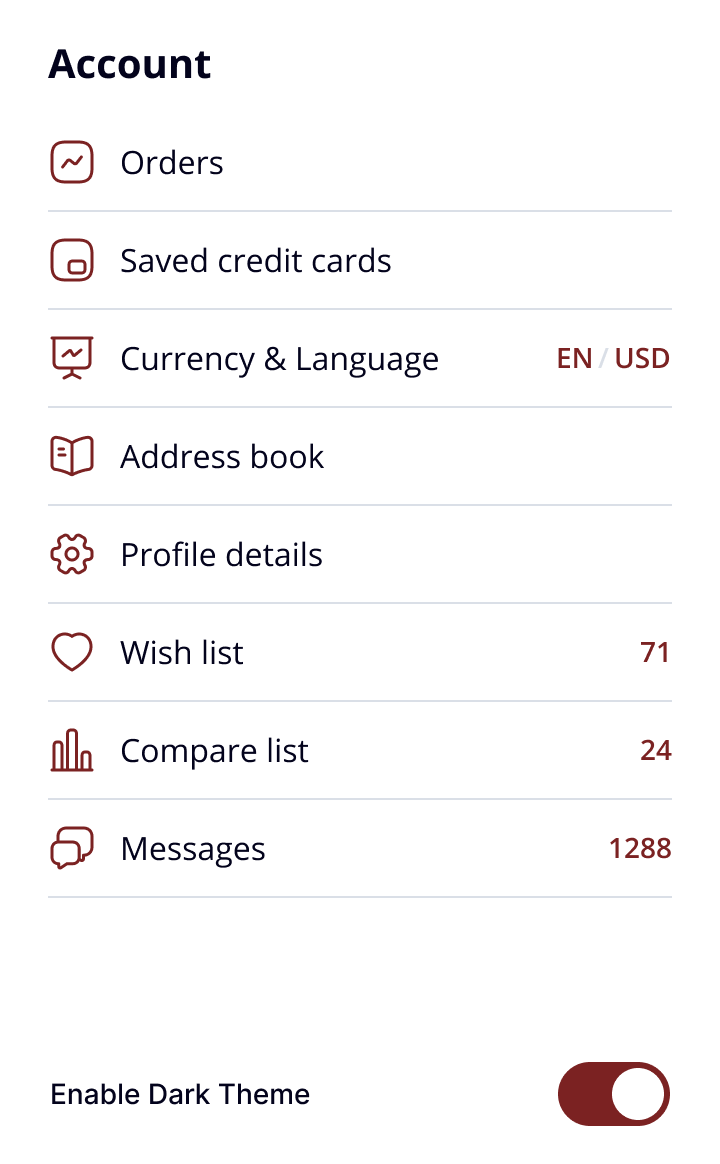"Displayed on a white, minimalist web page with black and gray text, this account dashboard features a bold black header titled 'Account' at the top. Directly beneath it, you can navigate various account management options organized in a vertical list, each accompanied by a simplistic, red, outline-style icon. Starting from the top, 'Orders' is paired with an ambiguous icon, followed by 'Saved Credit Cards,' represented by a clearer credit card icon. Below that, 'Currency and Language' is curiously illustrated by a projector screen icon, with current settings showing as 'English' and 'USD' on the right.

Continuing down the list, 'Address Book' is aptly symbolized by a book icon. Next, 'Profile Details' is somewhat mismatched with a sprocket icon, typically indicative of settings. For 'Wishlist,' a heart icon is placed to the left, showing 71 saved items. 'Compare List' is marked with a histogram icon on the left, noting the comparison of 24 items. Finally, 'Messages' displays a pair of thought bubble icons with a notification count of 1,288. Despite enabling the dark theme, the page remains in a white layout with minimalistic design, highlighting stark, almost rudimentary graphics."